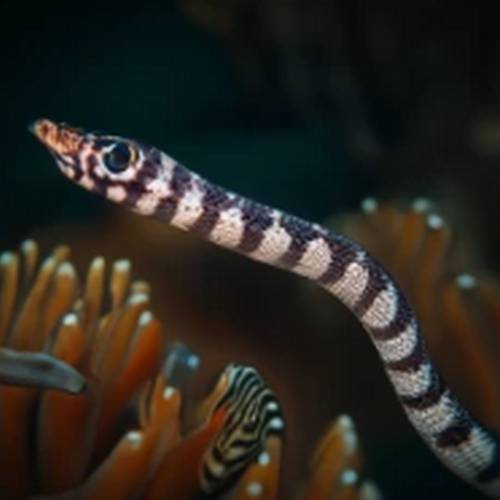This underwater photograph captures a striking scene featuring a sea snake with distinctive white and black horizontal stripes, emerging from the bottom right of the image and extending towards the center. The snake has a pointed snout with an orange-reddish hue and a large, round black eye, highlighted by a gray outline and a touch of yellow. The background, blurred and dark with shades of deep blue and green, suggests a submerged environment, populated by various sea plants. Prominent among these are large, orange sea plants with white tips, scattered to the right and bottom left of the image. One plant, in particular, features a white and black stripe pattern that matches the sea snake, suggesting an adaptation for camouflage. Additionally, there is a blurred black and white zebra-striped pattern towards the bottom center, possibly part of another marine creature, adding further intrigue to this underwater scene.